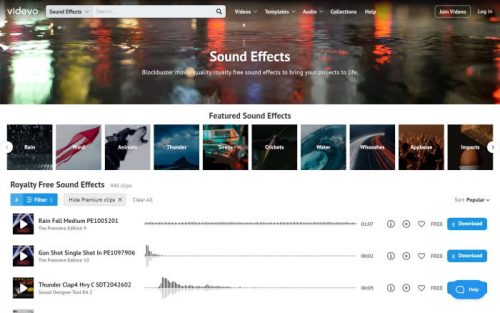This emergency webpage hosts a vast array of multimedia resources designed to assist users in times of need. On the right side of the page, there is a search field where users can easily look up specific sound effects. The navigation links include sections such as "Videos," "Templates," "Audio Collections," "Help," and an option to "Join Video." Additionally, users can log in to access more personalized features. The available sound effects cater to various scenarios and include categories such as rain, wind, thunder, crickets, water, wishes, applause, and impacts. Furthermore, there is a special section for reality-free sound effects featuring rainfall, medium impact sounds, gunshots (single shots), and thunderclaps.